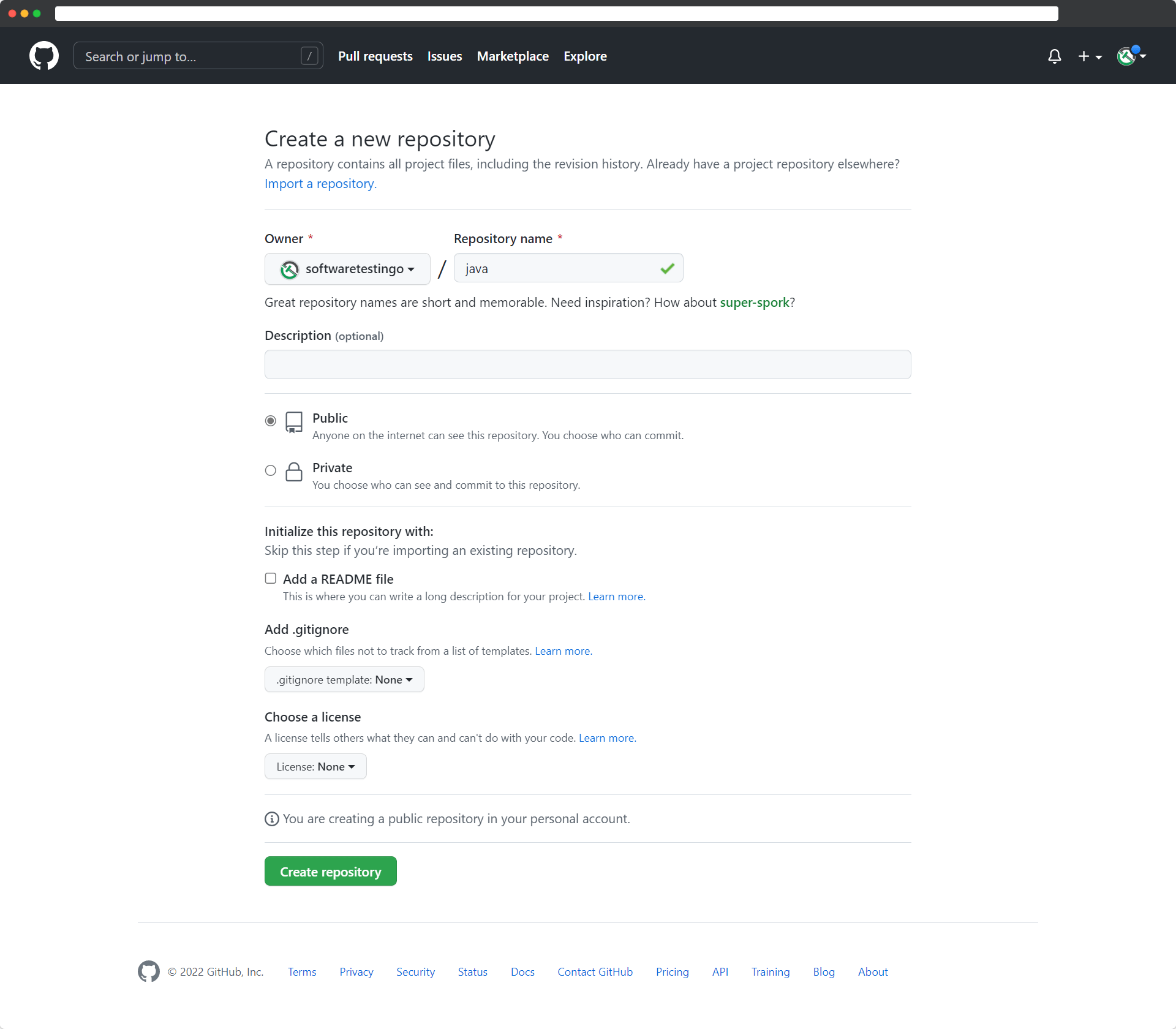The image appears to be a screenshot of an Apple application interface, specifically related to creating a new repository. The top section of the interface features a header strip with the recognizable three colorful dots (red, yellow, and green) on the upper left-hand side, which is typical of Apple applications for window control.

Directly below the header strip, there is a search field positioned on the left side of the interface. Beneath the search field, there are several navigation links that are challenging to read. The first link seems to state either "full reports" or "pull reports". Following that is a link labeled "Marketplace". The link between these two is indistinct and not easily decipherable.

The main area of the page is predominantly white and starts with a bold header that reads "Create a New Repository". Below this header, there are numerous actionable items and options for customizing the new repository. These options likely include input fields, dropdown menus, or checkboxes to define the repository's settings and preferences.

At the very bottom of the interface, there is a prominent green button labeled "Create Repository", which users would click on to finalize the creation of the new repository.